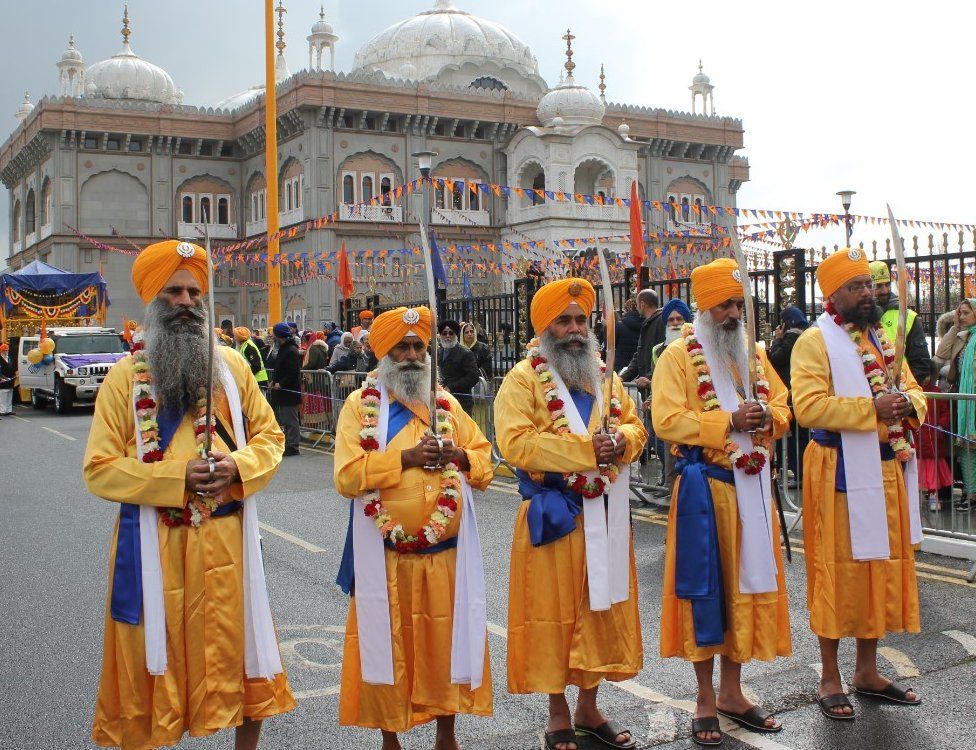In this photo, set against the backdrop of what appears to be an Indian or possibly Nepalese city, a group of five elderly gentlemen stand prominently in the foreground. They are all dressed in strikingly similar traditional attire: long orange tunics paired with long white scarves, and ornate orange turbans crowned with jeweled metal centerpieces. Each man boasts a long, bushy beard and mustache, contributing to their dignified yet somewhat disheveled appearance, and they are all wearing open-toed brown sandals. Around their necks hang vibrant floral wreaths made of blossoms in red, white, and different shades of yellow. They clutch swords in their hands, which are held closely in front of them, adding a regal yet imposing aspect to their look. Their attire also includes a blue sash attached at the waist, contributing to the colorful ensemble.

The scene unfolds on a street marked with yellow lines, suggesting a public or ceremonial space. To the right, a tall black fence, lined with spectators, stands behind a silver barricade, while others between the barricade and fence are adorned in colorful scarves. On the far left, a palace featuring multiple stories and domes with intricate cross-like finials serves as a majestic backdrop. The palace's architecture is adorned with long windows and has a flat roof dotted with blue and orange pennants. Further to the right, a truck decorated with balloons and an area with blue-tinted ornaments add to the festive atmosphere. The day appears overcast, casting a subdued light over the scene, hinting at a sober celebration that feels both contemporary and timeless.